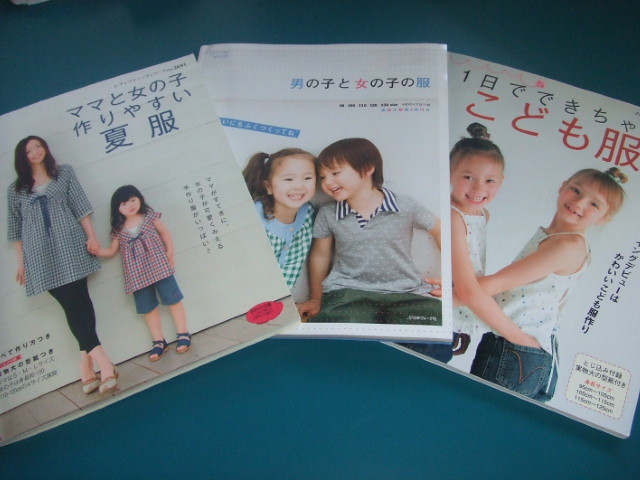In this photograph, three clothing pattern packages are displayed against a dark teal blue background, arranged in a slightly overlapping, fanned-out formation. The packaging, predominantly white, features a mix of Asian and Caucasian models and is adorned with Oriental-style typography indicating the titles. The pattern package on the left depicts a mother in her 20s and her young daughter, perhaps around four or five years old, both sporting a coordinated outfit of a top, black pants, and brown shoes for the mother, and blue shorts, blue sandals, and a blue and red top for the daughter. The center package showcases two children, around four years old, modeling clothes; a boy on the right wears a grey top with a black-striped collar, and a girl on the left sports a blue top with a green and white checkered pattern. The rightmost package features two girls, approximately five years old, each wearing sleeveless tops—one with white dots and the other with brown dots—paired with jeans, standing with their hands in their back pockets and their hair tied up, smiling and holding each other. The backdrop and surface on which these packages rest are a striking turquoise or dark teal, enhancing the vibrant and cheerful presentation of the clothing patterns.